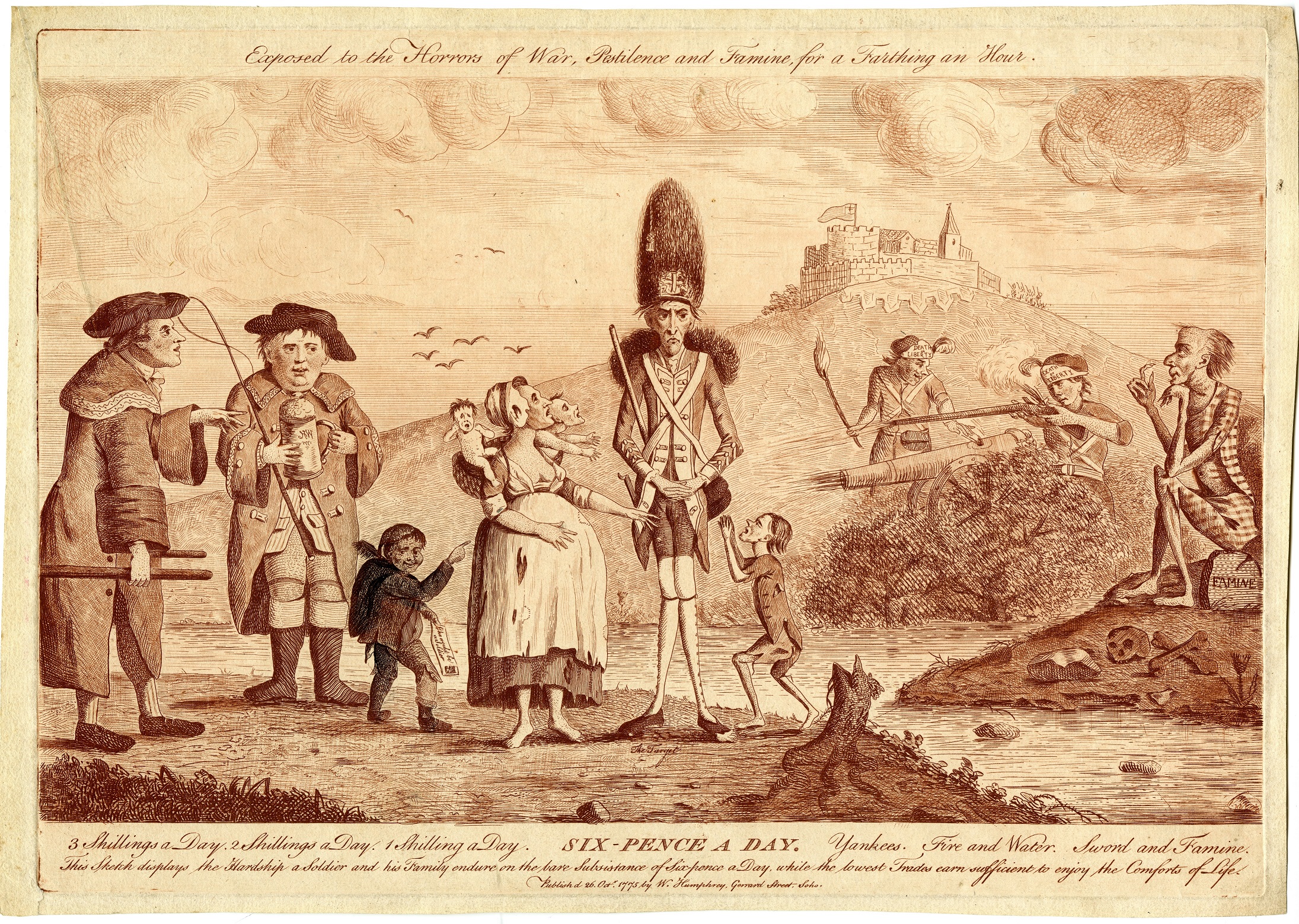In a sepia-toned, cream-colored background, the detailed drawing depicts a poignant scene, likely a piece of anti-war propaganda from the late 1700s or early 1800s. At the top, written in elegant script, is the phrase "Exposed to the horror of war, passing into famine." At the bottom, also in script, is "Six pence a day." Central to the composition is a tall, gaunt man wearing a headdress, symbolizing authority yet fraught with helplessness. Flanked by a woman in a white apron holding babies and begging children, the man's expression mirrors the surrounding despair. On the left, two British soldiers don flat-brimmed hats and period-specific attire, with one holding a whip or fishing pole, suggesting enforcement or a futile attempt at sustenance. To the right, a skeletal figure sits on a hill next to a body of water, evoking imagery of death and famine. In the far background, a castle-like fort stands ominously on a distant hill, while birds and seagulls punctuate the grim sky. The other scattered figures—soldiers carrying muskets and cannons, a fisherman gazing forlornly at the soldiers, and a man tugging a hand cart—collectively embody the collective suffering and despondency induced by war.